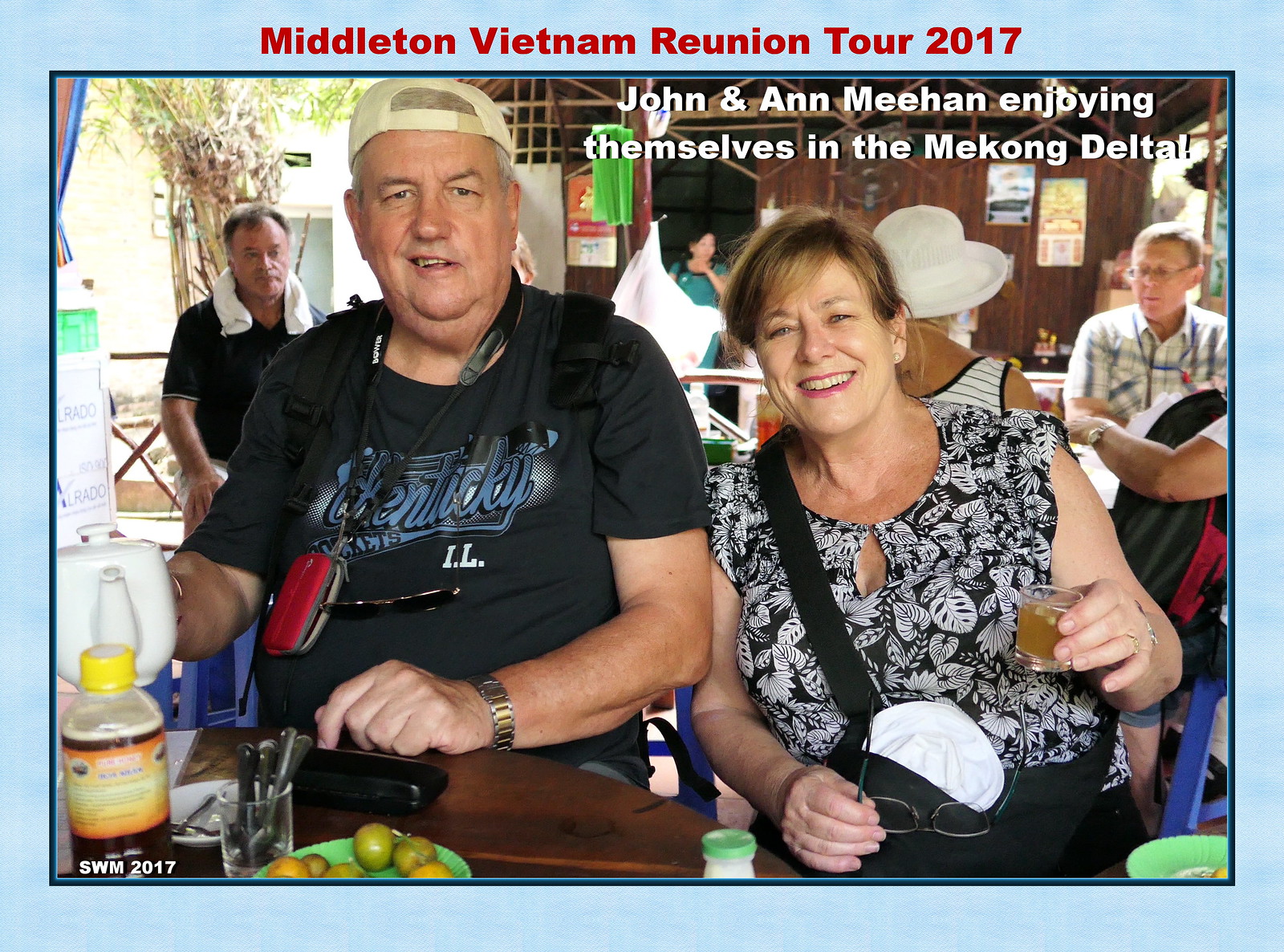The image, titled "Middleton Vietnam Reunion Tour 2017" in bold red font at the top, features a blue border and showcases John and Ann Meehan enjoying themselves in the Mekong Delta. They are sitting at a brown table, possibly in an outdoor café or restaurant that is covered but has an opening to the outside on the left. Ann Meehan, on the right, is smiling with brown hair and wearing a black and white floral shirt. She is holding a small bottle or glass containing a yellow liquid, which could be an alcoholic drink. John Meehan is seated next to her, casually dressed in a generic t-shirt, possibly white, and is wearing a white hat. In the background, multiple people can be seen, including a man in a black shirt with a towel around his neck, and another man with glasses and a white shirt engaged in conversation. On the table, there is a green bowl with some fruit and a bottle with a yellow label. The atmosphere suggests a leisurely gathering under a roofed area.